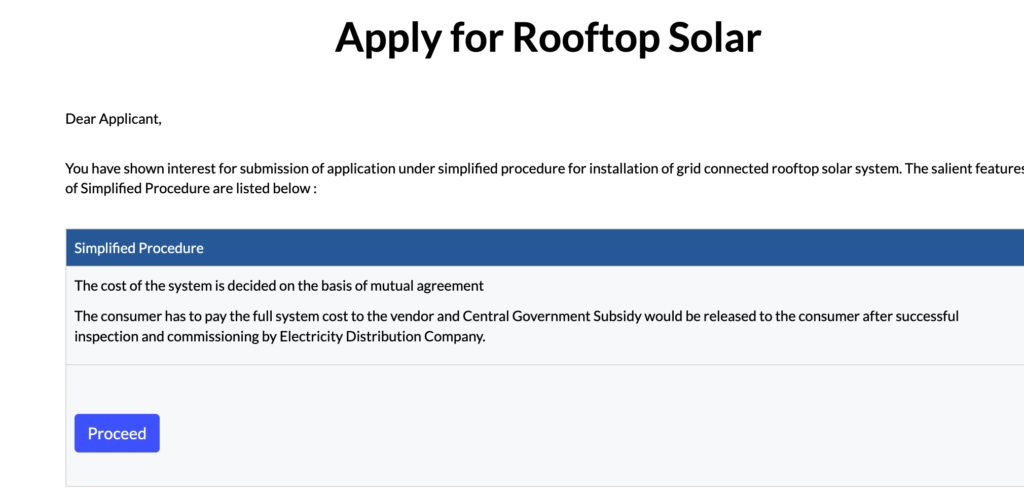Caption: 

An email titled "Apply for Rooftop Solar" is displayed, with the title written in bold black font size approximately between 14 and 18 points. The email begins with a formal address, "Dear Applicant," and states the recipient's expressed interest in applying for a grid-connected rooftop solar system under a simplified procedure. Below this introduction, a blue box with the heading "Simplified Procedure" in white letters highlights the simplified application process. Adjacent to it, a white box details the procedure: the cost of the solar system is based on mutual agreement, with the consumer required to pay the full system cost upfront to the vendor. A central government subsidy will be provided to the consumer after an inspection and commissioning by the electricity distribution company. The main body of the text, including "Dear Applicant" and the procedural details, is written in black font. At the bottom of the email, a prominent blue button labeled "Proceed" in white letters invites the recipient to continue with the application process.